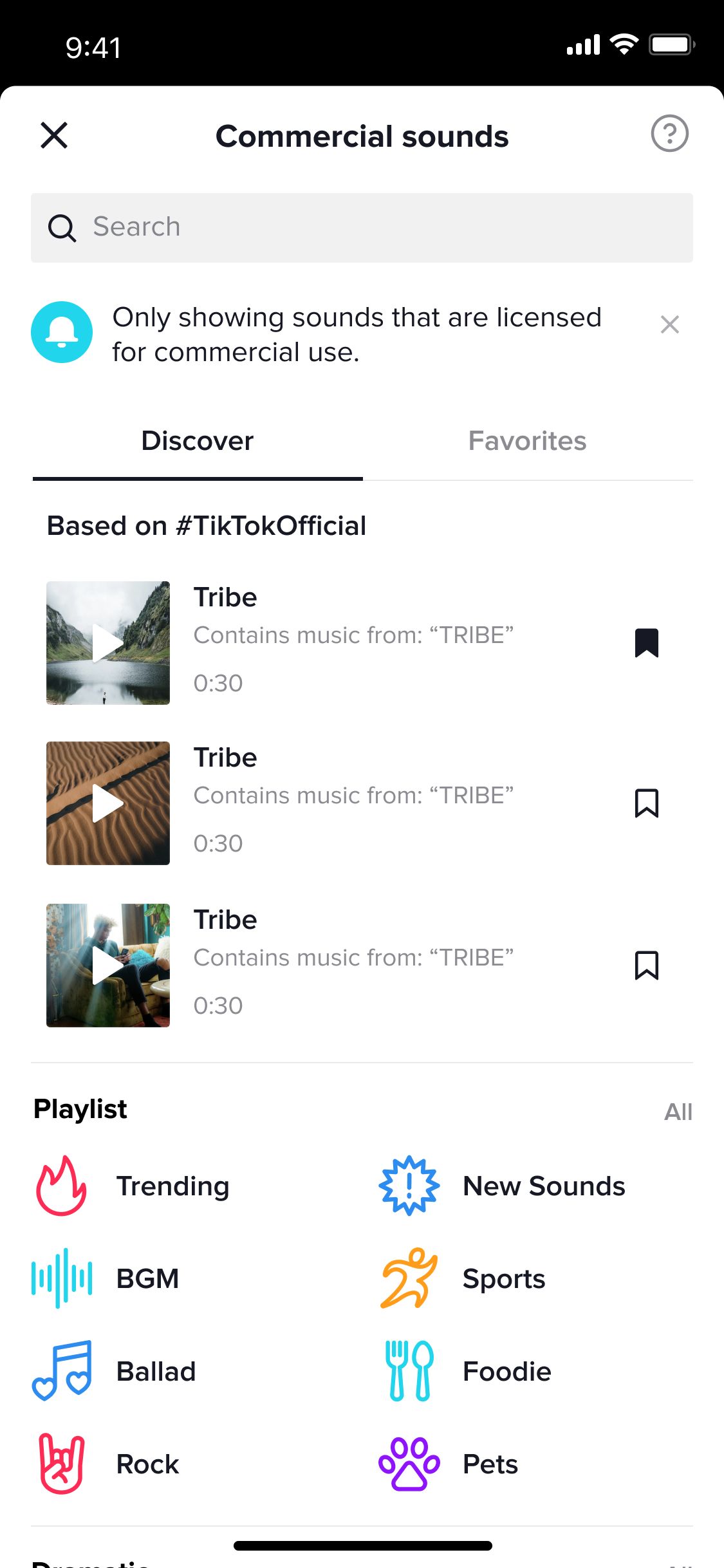This is a detailed screenshot of a mobile phone screen displaying a web page. At the top of the screen, there's a black status bar. On the upper left, the time is shown as 9:41 in white font. On the upper right, icons for mobile signal, Wi-Fi signal, and battery level are visible. 

Below the status bar, the web page begins with a predominantly white background. In the upper left corner of this section, there is a black "X" icon. In the upper right corner, there is a red circle with a red question mark inside it. Centered on the screen in bold black font is the title "Commercial Sounds."

Beneath the title is a gray search field with a black magnifying glass icon on the left side. The placeholder text in the center of the search field reads "Search." 

Below the search bar, there is a blue circle containing a white bell icon. To the right of this circle, black text reads, "Only showing sounds that are licensed for commercial use." Following this text, on the far right, there's a small gray "X."

Next, there are two tabs: "Discover" and "Favorites." The "Discover" tab is selected. Just below these tabs, a heading reads, "Based on hashtag TikTok Official." 

The content section displays three selections, each labeled "Tribe," with the description "Contains music from tribe." Each selection is 30 seconds long.

At the bottom of the screen, there is a white rectangle with additional options: "Trending," "New Sounds," "BGM," and "Sports."